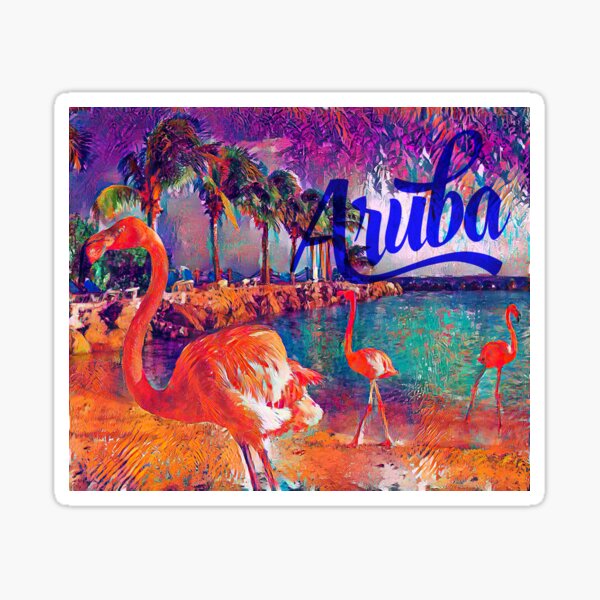The image depicts a vibrant and colorful oil painting with a distinct Miami Beach vibe, though the text "Aruba" is prominently featured in elegant blue calligraphy across the middle. The painting captures a lively beach scene at sunset or perhaps at night, filled with exaggerated, brilliant hues. In the foreground on the left, a striking pink flamingo stands poised on the bright orange-pink sand, drawing immediate attention. Two more flamingos, one in the middle and one to the right, appear smaller and further away, positioned along a curving beach that forms a gentle U-shape extending back to the right. The beach is lined with palm trees and, further along, rocky jetties and tables and chairs can be seen decorating the shoreline. The water is a surreal mix of neon green with deep purplish-blue tones, while the sky bursts with deep purple, magenta, and streaks of yellow. The palm trees themselves are unusually vibrant, adding to the eclectic and dazzling atmosphere of the painting. The entire scene is trimmed with a white border, enhancing the stark, vivacious contrast of the colors within.